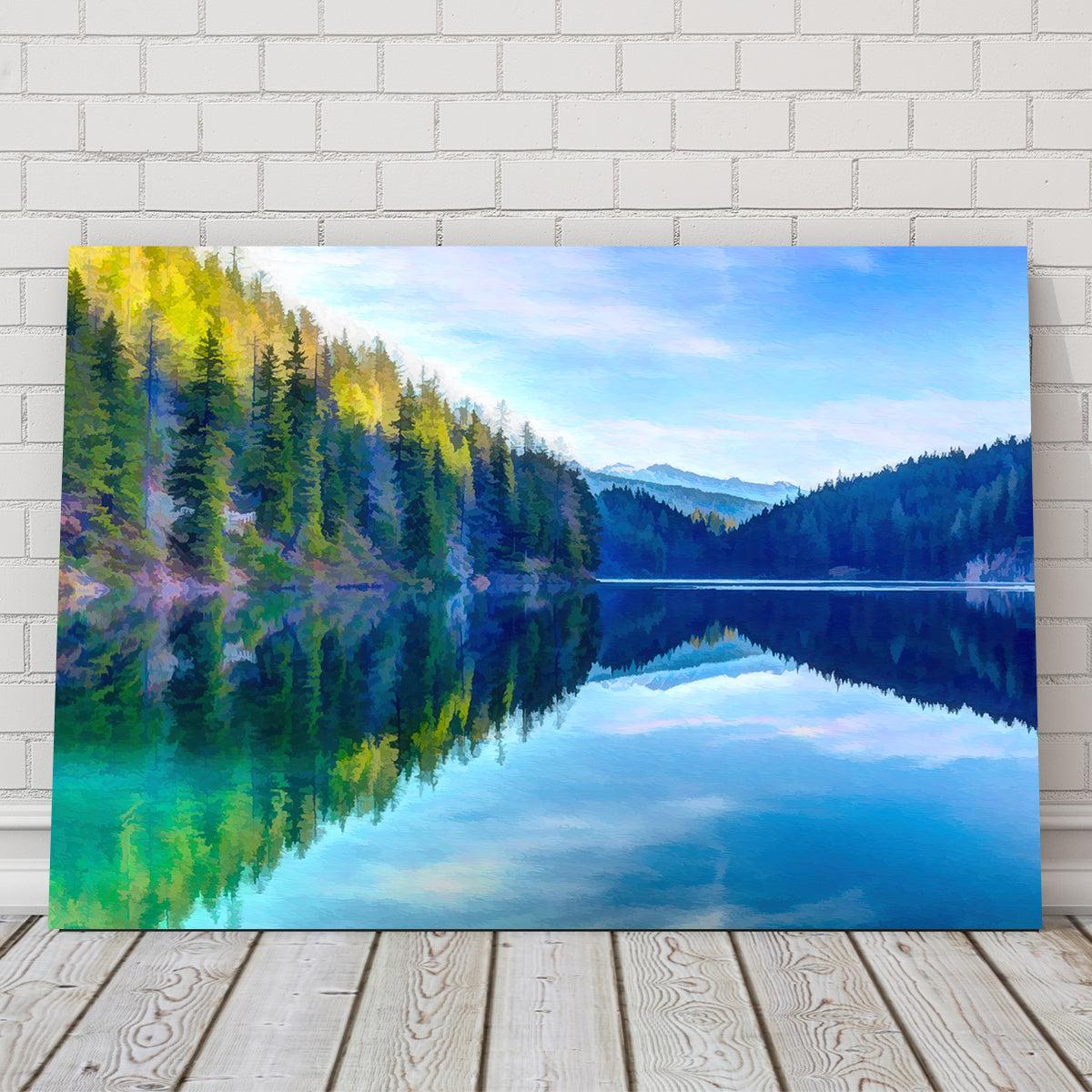The image captures a photograph of a painting displayed against a white brick wall, with a white-painted wooden floor in front of it. The painting, a large rectangular canvas that appears to be either watercolor or acrylic, depicts a serene mountainous landscape. The foreground features a tranquil lake, mirroring its surroundings with a strikingly clear and still surface. This mirror effect beautifully reflects the blue sky and wispy white clouds above, as well as the surrounding forest.

The scene is set during a time when the sun is low, casting a golden hue on the upper parts of the trees to the left. These trees exhibit a vibrant transition with bright yellow tips, transitioning into dark green shades and punctuated with touches of pink. Further left, a hill covered in green pine trees is bathed in sunlight, adding to the contrast. On the right side, the trees are shaded, appearing less green and more subdued in color.

In the backdrop, a majestic mountain range stretches across the horizon, some peaks capped with a hint of snow. The overall palette of the painting leans toward blue, likely due to shadowing effects and the calm, reflective water that dominates the foreground, capturing the essence of the peaceful, reflective moment in nature.